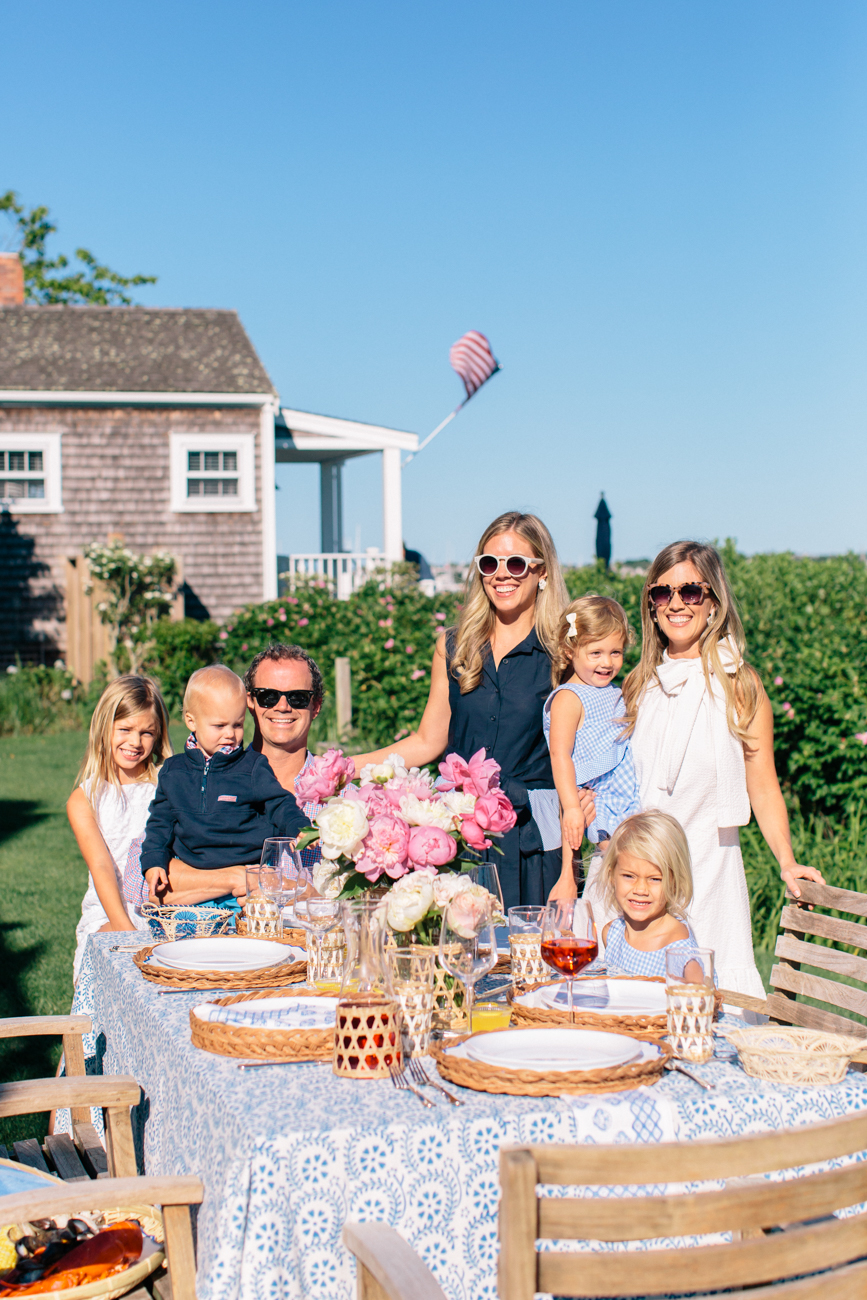A beautifully detailed photograph captures a cheerful family gathering, likely set outdoors in a lush green lawn, with a charming house in the background. The rectangular image highlights a rectangular table adorned with a white tablecloth featuring elegant blue vine designs. The table is meticulously set with round porcelain plates on basket-style placemats, surrounded by multiple light brown chairs. In the center of the table, a vibrant vase of red, pink, and white roses adds a pop of color. Assorted beverage glasses, including wine glasses, dot the table setup. 

The family members are dressed in a coordinated color scheme of blue and white, adding to the harmonious feel of the scene. Two women, each wearing sunglasses, stand on either side; the woman on the left is in a blue dress while the woman on the right holds a young girl and is dressed in white. Seated at the table is a man, also wearing sunglasses, with a young boy on his lap. Scattered around are three more children: a girl in blue close to the right woman, another girl in white near the left woman, and a girl in front to the right. 

The house in the background features classic brown shingles and has an American flag hanging from the porch, which hints at a setting reminiscent of Martha’s Vineyard. To the right, a white wooden fence adorned with climbing vines encapsulates the cozy, all-American atmosphere. Hedges with pink flowers further frame the scene, enhancing the picturesque quality of this family picnic moment.